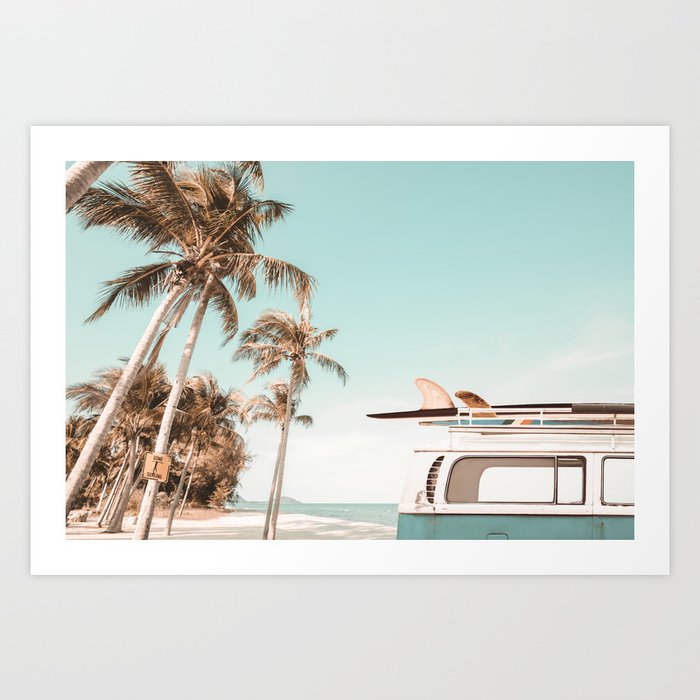The image is a rectangular photograph approximately 5 inches by 5 inches, set against a light gray background that forms a border. The photo itself has a thin, quarter-inch white frame and a subtle drop shadow, mimicking the style of a postcard. The scene captured in the photograph depicts a vintage VW van, its rear half visible in the lower right-hand corner. The van has a distinctive blue lower body and a white top with windows, adorned with surfboards lying on its roof. In the backdrop, tall palm trees sway in the beach breeze on the left side, amidst a sandy beach area that stretches towards a distant ocean. Overhead, the sky is a light blue-green, evoking a serene and coastal atmosphere. The entire composition has a slightly washed-out or overexposed quality, adding a nostalgic touch to the image.